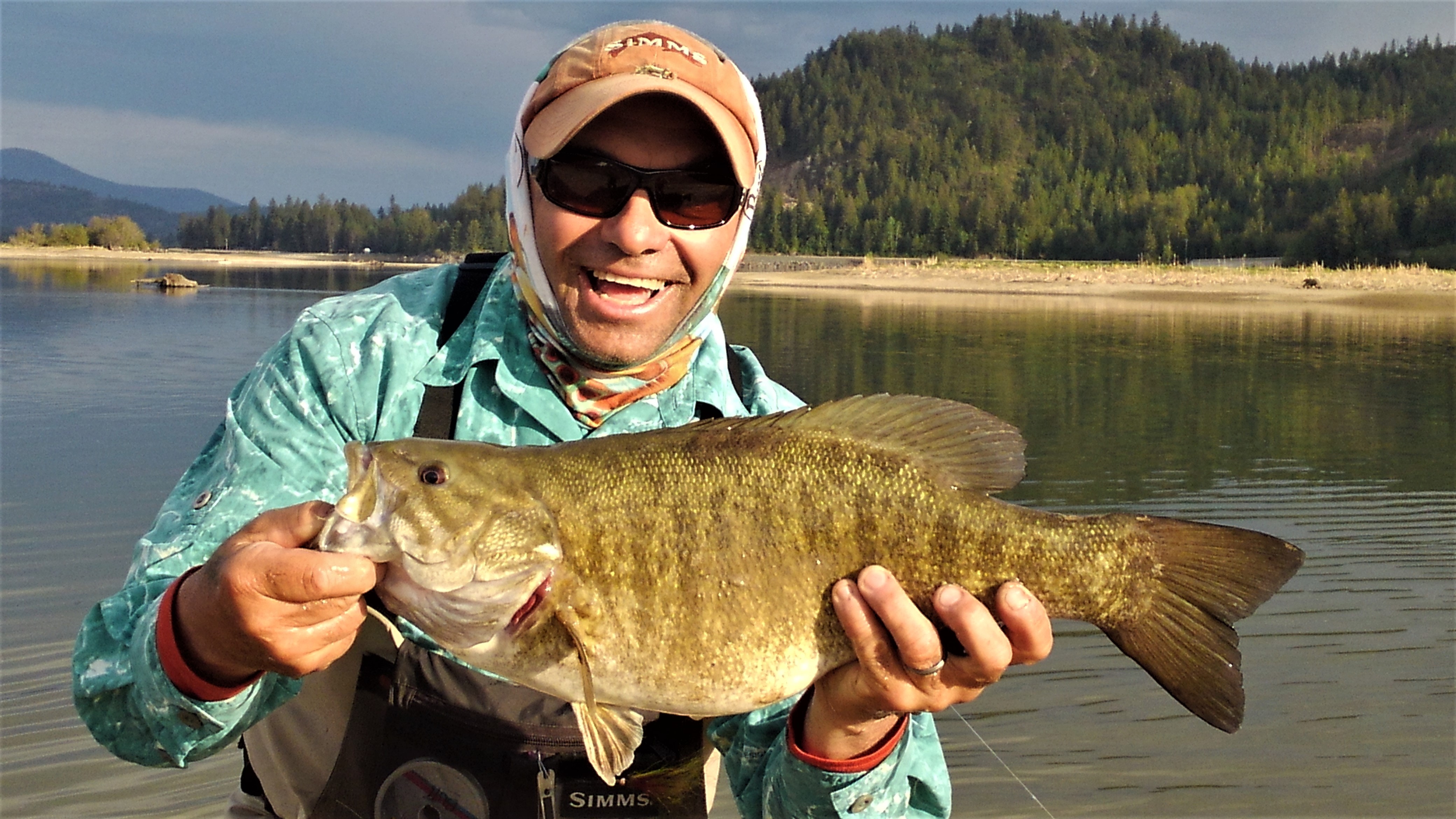The image captures an outdoor scene featuring a delighted fisherman proudly holding a large fish. The man, who is smiling broadly, sports sunglasses and wears a blue and white coat over layers of clothing suited for cold weather, including a light orange baseball hat with another cap or scarf covering it, and fish waders with "SIMS" written on them. Notably, he has a wedding ring on his left hand. In the backdrop, a serene lake stretches out to a small sandy beach, beyond which stands a lush landscape of tall pine trees with varying shades of green. The sky above appears light and dark blue, hinting at a mid-afternoon time frame. The scene suggests a possible location in the Rocky Mountains or near Washington State, enhancing the ambiance of an avid fisherman's successful outing in the great outdoors.